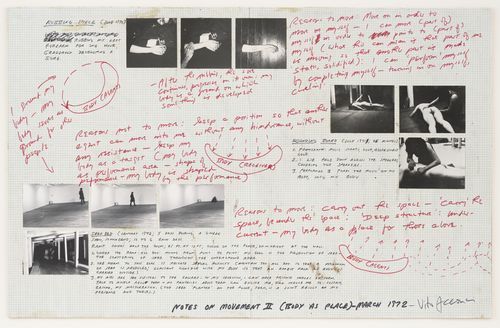The image is a landscape-oriented piece of conceptual art by Vito Acconci, titled "Notes on Movement 2 (Body as Place)," created in March 1972. It features a white grid paper background with extensive use of black and white photographs and red handwritten notations. Positioned across the top left are three black and white photographs depicting various parts of an arm. On the right side, three additional photographs show a person lying on their stomach with another person standing beside them, seemingly massaging their sides and back. In the bottom left corner, there are four more black and white photographs, depicting a figure engaging in different activities: standing against a wall, kneeling on the floor, and standing in a hallway. The red ink annotations, scattered around the images and black text, provide important information and context. The signature and a historical marking in the bottom left corner read, "March 1872," along with the words, "Notes on Movement 2". The overall visual gives an impression of a detailed research note with elements that evoke a sense of violence, horror, or clinical examination.